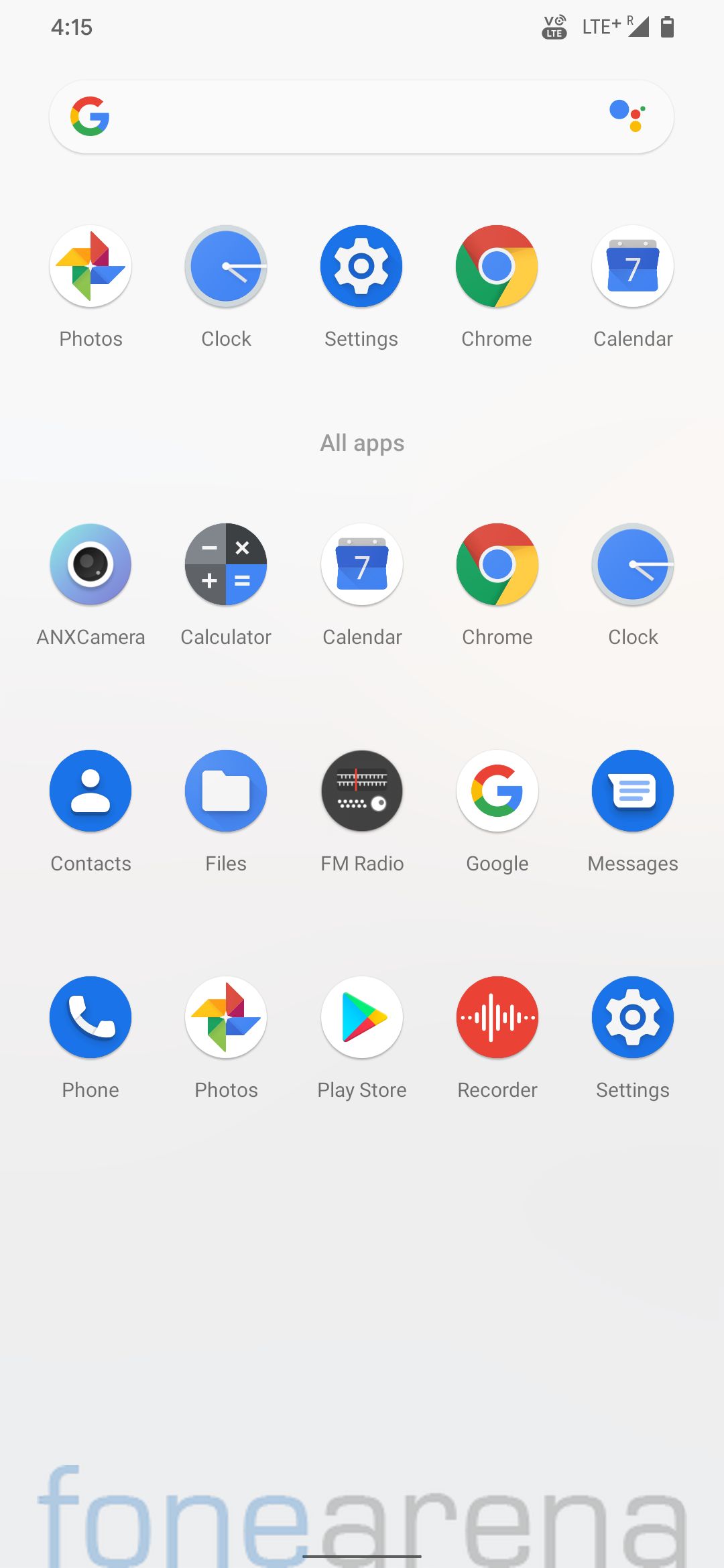Screenshot of a smartphone displaying various applications on a Google interface. The background is gray, and the time at the top left reads 4:15. On the right-hand side, indicators for LTE+ broadband connection and battery capacity are shown.

Just below, a search bar features the Google logo in red, yellow, green, and blue on the left, and a circular icon with a person symbol on the right. Below the search bar, several rows of application icons are neatly arranged.

The first row includes:
1. Google Photos - represented by a multicolored pinwheel.
2. Clock - displaying a blue clock face with white hands.
3. Settings - shown as a blue circle with a gear icon.
4. Chrome - depicted as a circle bordered in green, red, and yellow with a blue center.
5. Calendar - illustrated by a white icon with a blue calendar displaying the number 7.

The second section is labeled "All Apps" and starts with:
1. ANX Camera.
2. Calculator - a circle featuring plus, minus, equals, and multiplication symbols.
3. Calendar - same as the one in the first row.
4. Chrome - same as the earlier mentioned icon.
5. Clock - same as the previous clock icon.

The second row of apps includes:
1. Contacts - a blue circle with an outline of a head and torso.
2. Files - represented by a white file icon on a blue circle.
3. FM Radio - displaying a black radio dial with markings and a tuner line.
4. Google - a white circle with the multi-colored Google "G".
5. Messages - illustrated by a blue circle with a white paper piece icon.

In the final row:
1. Phone - a blue circle with a handset icon.
2. Photos - same multicolored pinwheel as mentioned earlier.
3. Play Store - represented by a white circle with a right-facing triangle.
4. Recorder - depicted as a red circle with sound wave illustrations.
5. Settings - same blue circle with a gear icon as previously noted.

At the bottom of the screen, the text reads "Phone Arena" in blue and gray font.